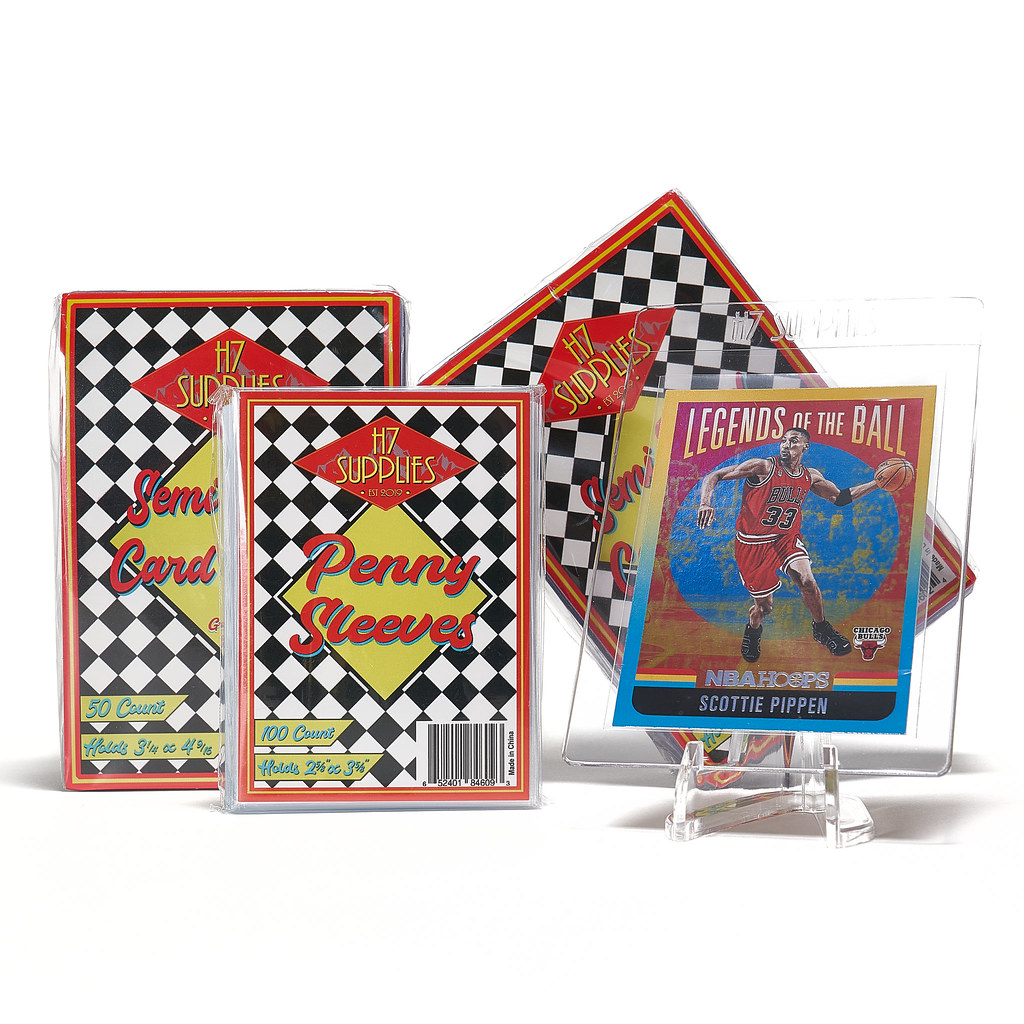The image shows a well-arranged display of basketball memorabilia and protective card sleeves against a pristine white background, likely set in a light box to enhance clarity. At the center, three packs of H. Evans Supplies (or H7 Supplies) Penny Sleeves are prominently positioned. The middle packaging shows a 100 count, labeled within a black and white checkered design bordered in red and yellow. The package's design features a retro diner-style script, reading "H. Evans Supplies Penny Sleeves," with the exact dimensions partially obscured. To the left, there's a smaller 50-count pack, similarly designed but more compact, giving a slightly clearer view of the red header and yellow diamond-shaped label. Behind these, a third pack is visible, slightly tilted, hinting at another size, though the specifics are hidden from view.

Towards the right, the image showcases a collectible basketball card encased in a protective plastic holder. The card is titled "Legends of the Ball," featuring Scottie Pippen of the Chicago Bulls, easily identified by his red jersey with the number 33. The card's design includes a striking gold and blue background, with a red banner displaying "Legends of the Ball" in gold lettering. The player is shown mid-action, running with a basketball, with "NBA Hoops" branding below his name. The entire scene suggests a promotional setup, perhaps an advertisement aimed at collectors, highlighting both the protective sleeves and the prized card. The vivid colors of black, white, red, yellow, green, light blue, tan, and gold dominate the image, creating an eye-catching visual display.